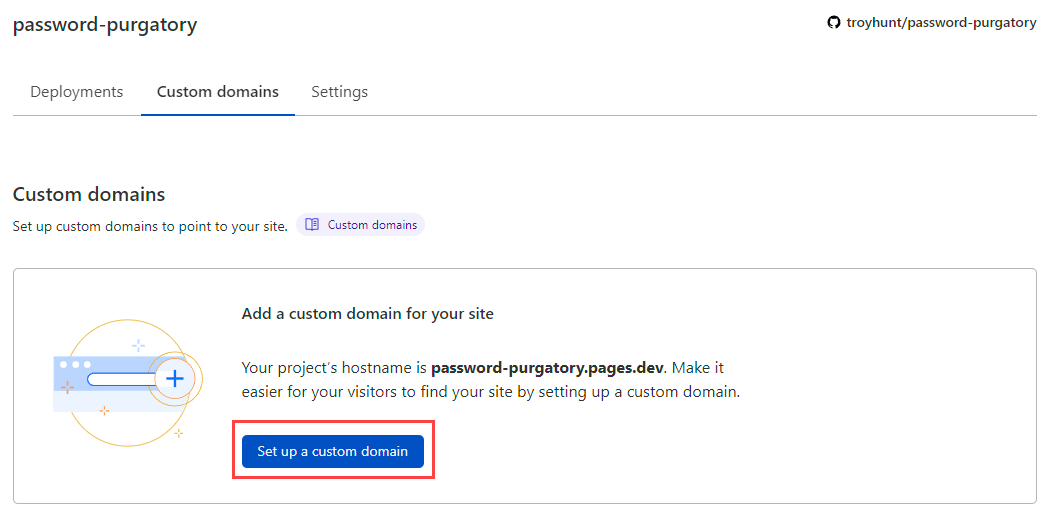This image depicts a GitHub page titled "password-purgatory." On the top right, there's a recognizable symbol, while the top left features the GitHub mascot, the "Octocat." The username displayed is "troyhunt-password-purgatory," indicating the owner of the page. Beneath the username, three tabs are visible: "Deployments," "Custom Domains," and "Settings," separated from the rest of the content by a thin, gray line. The "Custom Domains" tab is highlighted with a blue underline, showing it is currently selected.

The section below the tabs is dedicated to setting up custom domains for the site. The heading reads "Custom Domains - Set up custom domains to point to your site." Following this, there is a large rectangular button labeled "Add a custom domain for your site." The accompanying description provides more details: "Your project's hostname is password-purgatory.pages.dev. Make it easier for your visitor to find your site by setting up a custom domain."